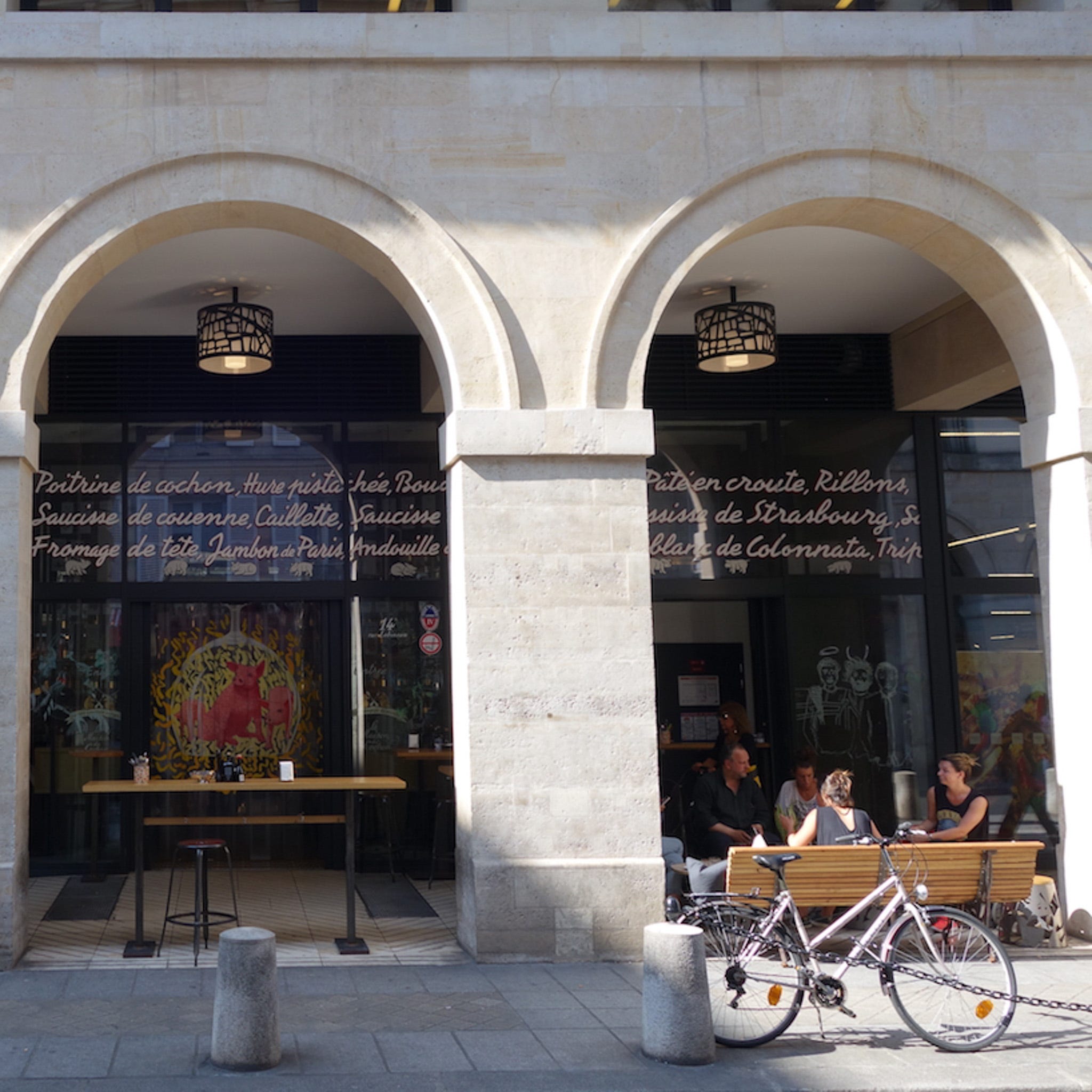The color photograph, taken in a square format, depicts the exterior of a European coffee shop, likely located in France, as indicated by the French text on the windows. The storefront features two large arches made from cream-colored stone, providing a covered seating area. On the left, there's a wooden bar rail supported by a steel bracket, accompanied by a table and a stool with a wooden seat. On the right, several people are seated on a wooden bench with a steel bracket, engaged in conversation.

The sidewalk in the foreground is styled with big square tiles and concrete bollards connected by a black chain, preventing car parking. A bicycle is parked with its kickstand engaged against one of these bollards and partially visible on the lower right of the image.

The shop itself has a glass front, and in the window, a pink pig figurine suggests an element of the cafe's branding. Inside the arches, round light fixtures hang from the ceiling, adding to the inviting atmosphere.